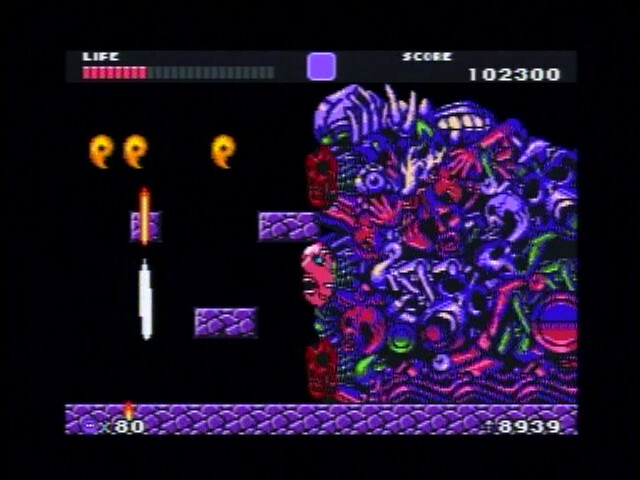A screenshot from a retro-style video game reminiscent of Super Mario World, but featuring unique creatures and vibrant colors. The scene is set in a 2D side-scrolling world with a completely black background, bringing focus to the game elements. The ground is depicted as a long rectangular strip mimicking rocky cave terrain.

On the right side of the image, there is a large, composite creature that seems to be a boss. This monster is composed of numerous smaller parts, displaying approximately ten distinct faces in various shapes and neon hues, including dark blues, purples, violets, pinks, greens, and reds. Intricate detailing shows faces and possibly limbs or other objects emerging from its mass.

At the bottom left corner, a fire symbol precedes the text "X80," while the bottom right corner displays the number 8939 in white next to another symbol. To the left of the giant creature are three staggered platforms that match the texture of the ground beneath.

Additionally, the image features small flame symbols moving either towards or away from the large mass, against white and orange lines. At the top left corner is a life bar indicating the player has taken significant damage, accompanied by the word "Life" in white text. Centered at the top, there is a lavender square, followed by the word "Score" in white letters on the top right, with a displayed score of 102300.